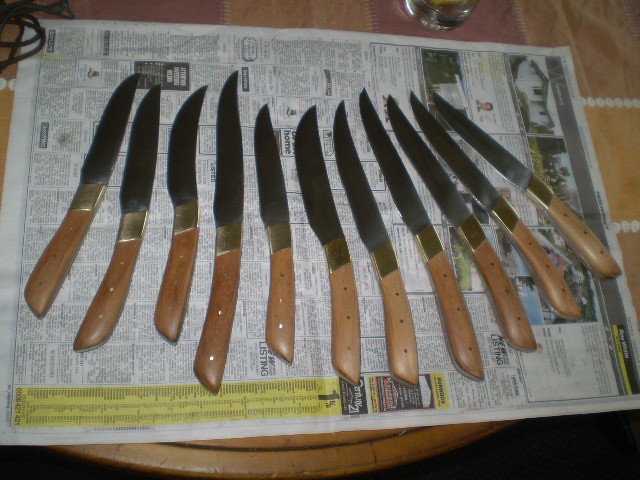The photograph captures a set of roughly 10 to 11 vintage-looking kitchen knives meticulously arranged on a piece of newspaper atop a tablecloth patterned with orange, pink, and white squares. The table itself is wooden and round, adding a rustic vibe to the scene. The knives, which are primarily steak and paring sizes, feature light brown handles, each secured with three silver screws and accented by golden rectangular metal elements before the blade. The blades vary, with some being straight and others curved. Surrounding the setup, the image includes hints of a clear glass, a piece of black cording, and other miscellaneous items, enhancing the candid, eBay listing-like appearance of the display.